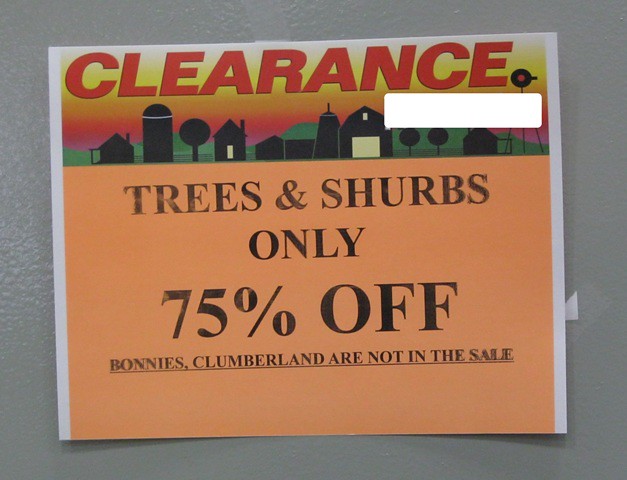This color photograph captures a sign taped onto a gray painted wall, promoting a clearance sale for a local company. At the top of the sign, bold red text announces "CLEARANCE." Just below this, a black silhouette illustration features a stylized farm scene, complete with barns, trees, and a grain silo. The background shifts to a light orange or pinkish hue where black text states, "Trees and Shrubs only 75% off." Notably, "shrubs" is misspelled as "shurbs" on the sign. A final line, underlined for emphasis, clarifies that "Bonnie’s, Clumberland are not in the sale." The sign appears to be taped at the edges, with visible tape on the right side, affixed to the gray wall.